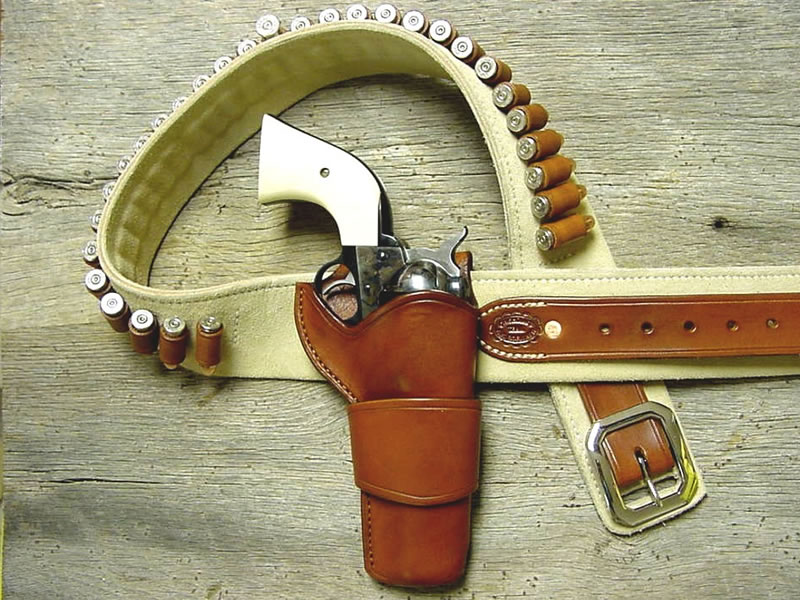The photograph features a detailed, classic gun belt setup meticulously laid out on a weathered, gray barn-wood surface. The centerpiece is a tan leather belt, adorned with brown leather accents and matching holster. The belt is intricately designed with approximately 30 or more bullet loops, each snugly holding a bullet, illustrating its utilitarian functionality and rugged charm. The holster, crafted from brown leather, contains a silver revolver featuring elegant ivory-colored grips. The belt's silver buckle, reinforced with brown leather straps, adds to its robust appearance. The entire setup, from the bullets to the leather craftsmanship, showcases a blend of durability and classic Western style, all highlighted against the barn-wood background.